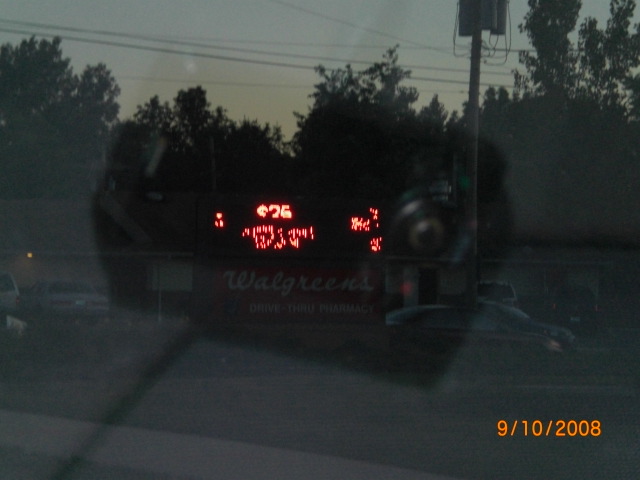The image captures an older-style Walgreens storefront, designed with a distinctive ranch house aesthetic. Taken in the evening, the sky is transitioning to darkness, casting a subtle twilight glow over the scene. The photograph appears slightly blurred, likely due to it being shot through a car window, which also produces a reflective glare. Centrally within the reflection, you can discern a faint outline of a camera, accompanied by the partial image of a metal button to its right. Notably, the bottom right corner of the image is timestamped with the date "9-10-2008," lending a nostalgic touch to this snapshot of a bygone era.